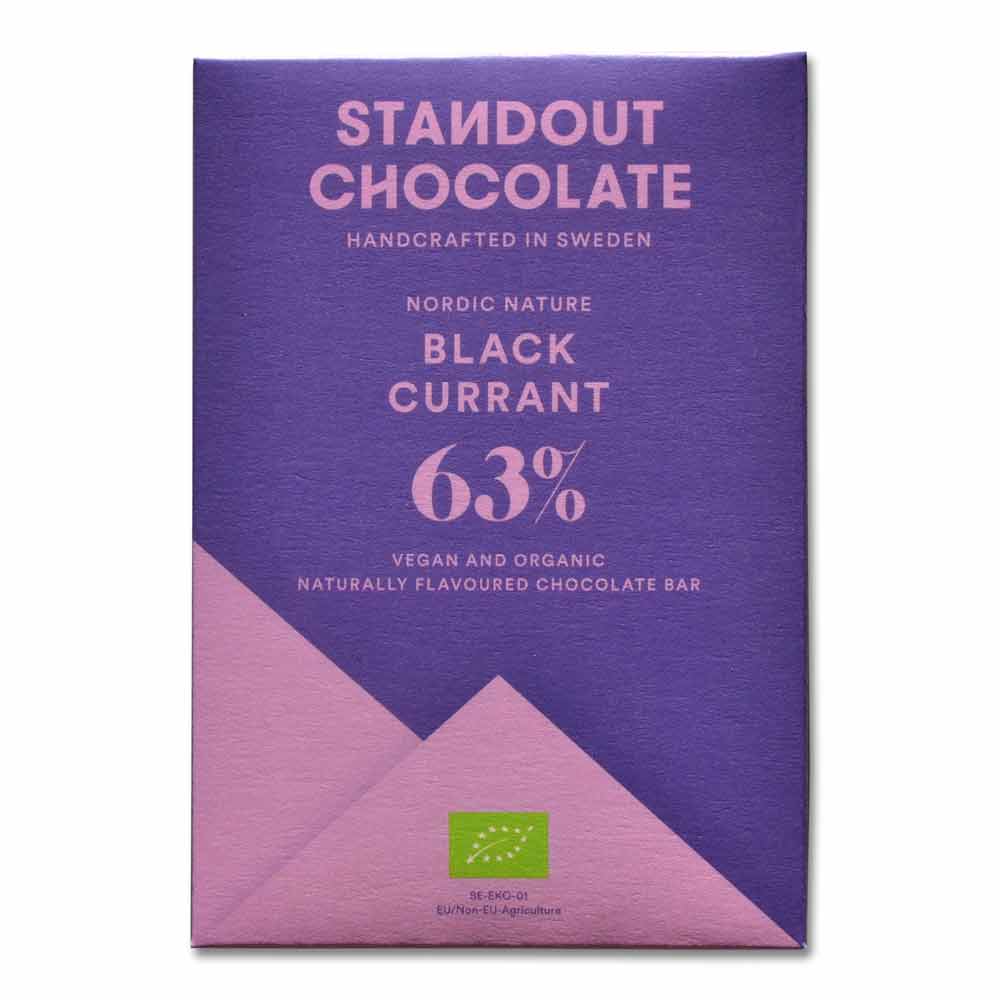This photograph features the front of a chocolate bar package that is taller than it is wide. The wrapper's predominant colors are purple and pink, with the majority being purple and the bottom section featuring a triangular, envelope-like pink design that points upward. The top portion displays the brand name "Stand Out Chocolate" in bold lettering with a distinctive backwards 'N.' Just below, it reads "Handcrafted in Sweden," followed by "Nordic Nature, Black Currant 63%," and "Vegan and Organic, Naturally Flavored Chocolate Bar." A motif of triangles in matching purple supports the pink bottom section. Additionally, there is a small green flag with a leaf stenciled below it, accompanied by the text "SCEKO-01, EU/non-EU agriculture."